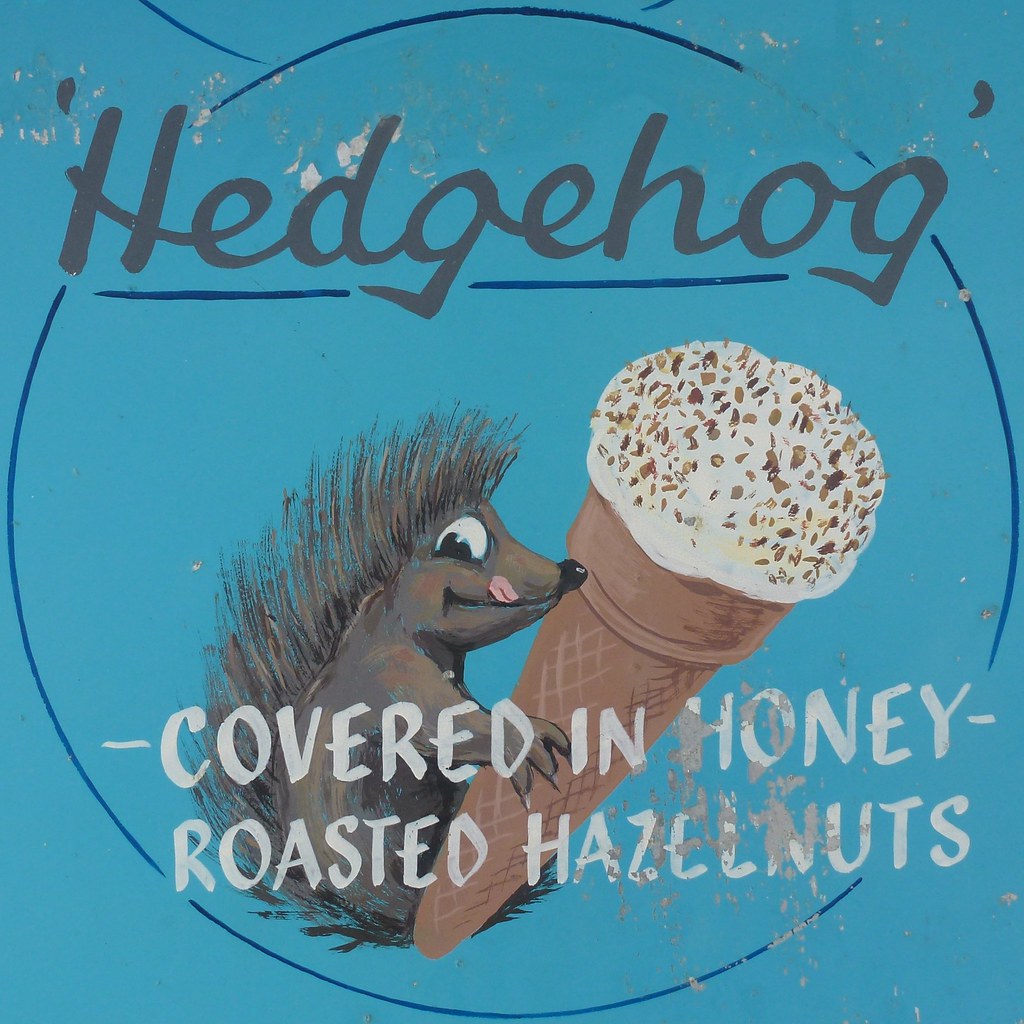The image depicts an old, weathered advertisement painted on the side of a light blue exterior wall. Significant portions of the blue paint have chipped away, revealing the white and grey concrete underneath, giving the scene a rustic feel. At the center of the image is a thin, darker blue circular line enclosing the text "Hedgehog" written in large, cursive grey letters at the top. Below this text, a charming cartoon-like hedgehog, brown with visible spines on its back, smiles broadly with its tongue sticking out, its wide, bright eyes looking to the right. The hedgehog holds a large brown ice cream cone with a white scoop of vanilla ice cream, adorned with little brown cylinders and squares suggesting various toppings. Superimposed over the hedgehog and the ice cream cone are the words "covered in honey roasted hazelnuts," also in grey. The overall hand-drawn, hand-painted nature of the advertisement combined with its age and condition evokes a sense of nostalgia.